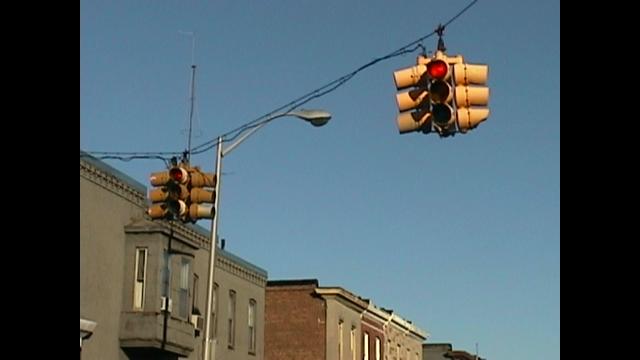This color photograph captures a clear, cloudless blue sky as the backdrop for two red traffic lights suspended from a single black wire. The wire originates from the top right of the image and continues toward the left until it meets the first traffic light. From there, an additional wire extends to the second traffic light, which is also lit red. Both traffic lights are of the traditional yellow design, featuring red, yellow, and green lights. 

Beneath the traffic lights, a tall, chrome-colored streetlight stands, featuring an arm that extends out with an unlit lamp at the end, resembling a black bowl. Behind the streetlight are the tops of several old-timey buildings, hinting at architectural styles possibly dating back to the 1930s to 1960s. The foremost building is gray with tall, thin windows that have black bottoms and white-topped shades, and it features a small alcove with surrounding windows and a green roof adorned with a design underneath. In the background, a small black chimney rises, though it is unclear which building it belongs to.

Adjacent to the gray building is a brick structure distinguished by a front section flanked by two concrete-colored projections. This brick area showcases tall windows and a decorative flared top that mirrors the front's proportions. Thin cables or wires descend from the background, creating a vague triangular formation, possibly connecting to the main wire. 

On either side of the photograph, thick black vertical bars frame the image, providing a sense of balance while emphasizing the central elements. Notably absent from the scene are any people, animals, plants, or vehicles, leaving the focus squarely on the architectural features and the suspended traffic lights.